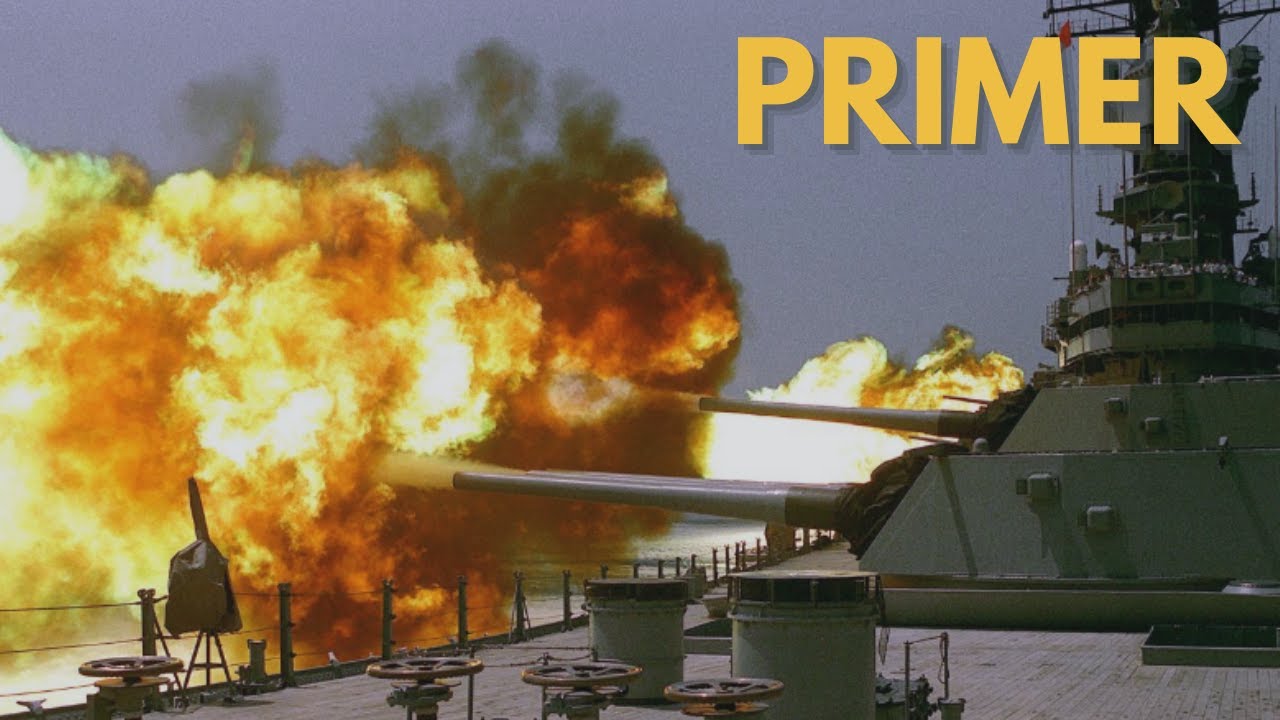This is a photograph of a military battleship, captured in a dramatic moment as its cannons fire to the left of the frame. The ship, painted in olive green, features prominently against a backdrop of a clear blue sky. In the upper right corner, the word "Primer" is emblazoned in bold yellow text. The battleship's control center, also painted olive green, is visible below the text. The deck, a mix of gray and dark gray surfaces, is devoid of any crew members but shows controls such as steering wheels used to open valves. The cannons, extending out to the left, emit a powerful and fiery explosion with vivid red, orange, and yellow flames intermixed with dark gray smoke. The explosion creates a striking visual contrast with the serene blue sky. Below the cannon's firing position, a fence marks the edge of the deck, where faint traces of water are visible. The overall composition is so tight and detailed, it almost appears like a 3D model or animation.